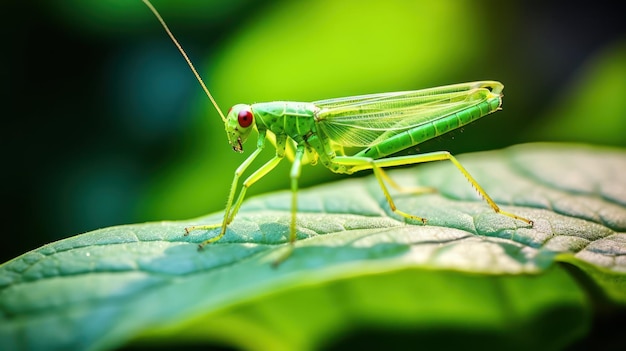This vibrant outdoor close-up photograph captures a green grasshopper perched on a large green leaf that occupies the center of the frame. The grasshopper's elongated body is adorned with dark green spots and features a pair of long, thin translucent yellow wings. The insect, oriented towards the left, has six spindly legs—lighter in color, almost yellow—and appears to be in perfect health except for the absence of one antenna. The remaining antenna is long and yellow. Notably, the grasshopper has striking red eyes with black pupils, prominently positioned at the sides of its head. Beneath the eyes, its small but visible black mandibles are poised. The background consists of an out-of-focus array of greens, blues, and blacks, providing a stark contrast to the leaf's and grasshopper's bright colors and adding depth to the image's composition.